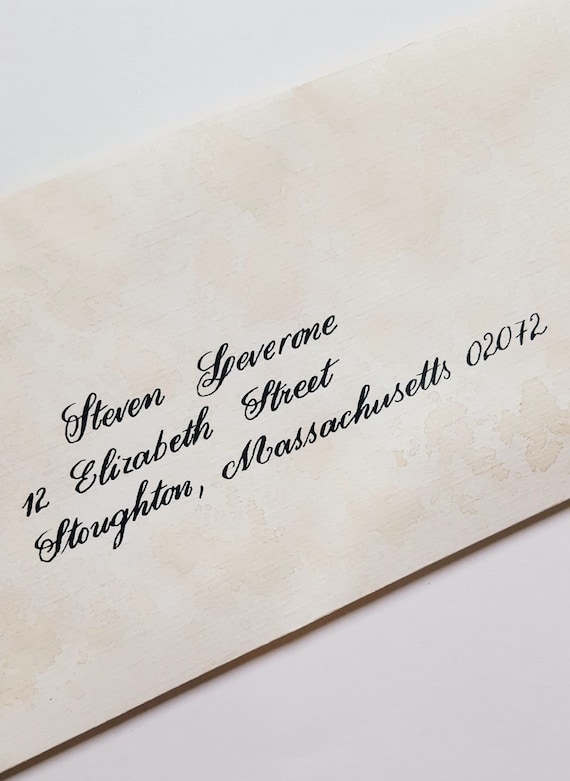This image depicts a close-up of a beige envelope resting on a white background. The envelope features a design with faded brown and pinkish stain-like blotches, resembling an artistic, vintage effect rather than actual stains. Addressed in an elegant cursive font, the text on the envelope reads "Stephen Leverone, 12 Elizabeth Street, Stoughton, Massachusetts, 02072," with the state name fully spelled out. The envelope lacks a stamp and any other markings, highlighting its pristine condition against the contrasting white surface.